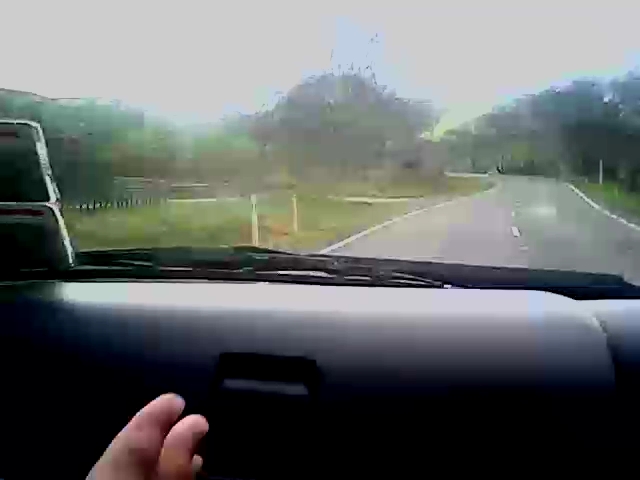This image captures the first-person view from the passenger seat of a vehicle moving down a two-lane asphalt road, lined with white striped lines and surrounded by grassy areas. The grainy, pixelated quality of the photo suggests it was taken with an old cell phone, making it quite blurry. The foreground prominently features a portion of the dashboard, including the glove box handle, while part of the windshield wiper is visible on the windshield. Two stickers are affixed to the left side of the windshield glass. In the bottom left corner, the tips of three fingers—likely the index, middle, and ring fingers—are just visible. Outside the windshield, you can see the road stretching ahead, flanked by trees on both sides. Two poles are positioned in the grassy area on the left, indicating a driveway entrance. The sky appears gray and hazy, adding to the overall indistinct clarity of the scene.